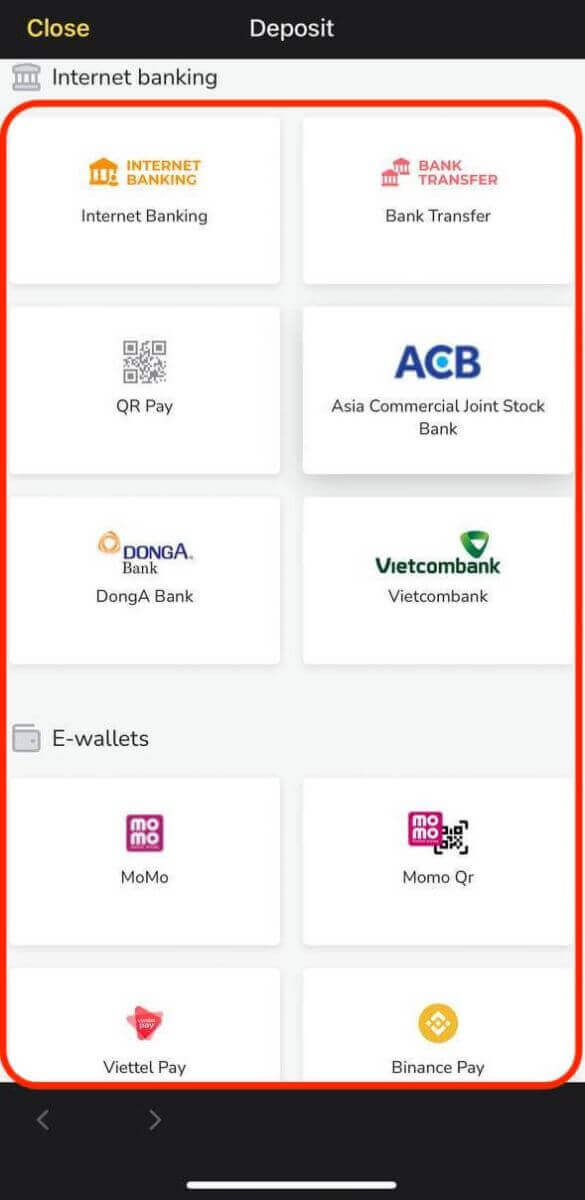This is a screenshot from an unidentified digital interface. At the top, a black banner features the words "Close" in yellow letters and "Deposit" in white letters. Below the banner, the background of the interface is predominantly white. 

An icon resembling a building is labeled "Internet Banking." Beneath this, a red vertical rectangle encases several categories and options under "Internet Banking," including:
- Internet Banking
- Bank Transfer
- QR Pay

Listed banks include:
- Asia Commercial Joint Stock Bank
- Donga Bank (spelled as D-O-N-G-A, with a capital D and A)
- Vietcom Bank

Following the bank listings, the category "E-wallets" is presented, featuring:
- Momo (spelled as M-O-M-O, with capitals on the M's)
- Momo QR
- Viettel Pay (spelled as V-I-E-T-T-E-L, with all capitals)
- Binance Pay (spelled as B-I-N-A-N-C-E, with all capitals)

The interface appears primarily text-based, with no photographs, people, animals, plants, or trees. The image is notably taller than it is wide.